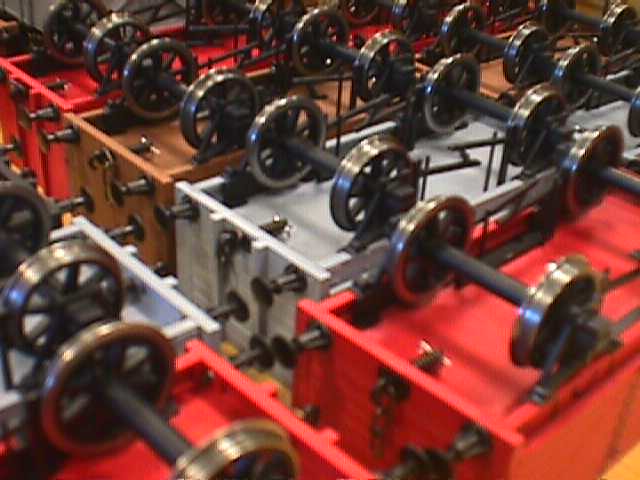This digital indoor photograph showcases numerous upside-down toy train boxcars arranged in rows extending diagonally from the upper left to the lower right. The cars feature metal stoppers at their ends, designed to prevent them from colliding when connected. The cars predominantly appear to be made of plastic with colors following specific patterns: the bottom right row transitions from red to white. The subsequent row follows a red, white, orange, and red sequence, with similar patterns in the upper right area. Complementing these colors, additional cars in brown and light blue are also visible. Each car is equipped with a set of four wheels, likened to barbells, attached to what would be the top side if they were right-side up, adding to the intricate detail and inviting curiosity about their function and design.